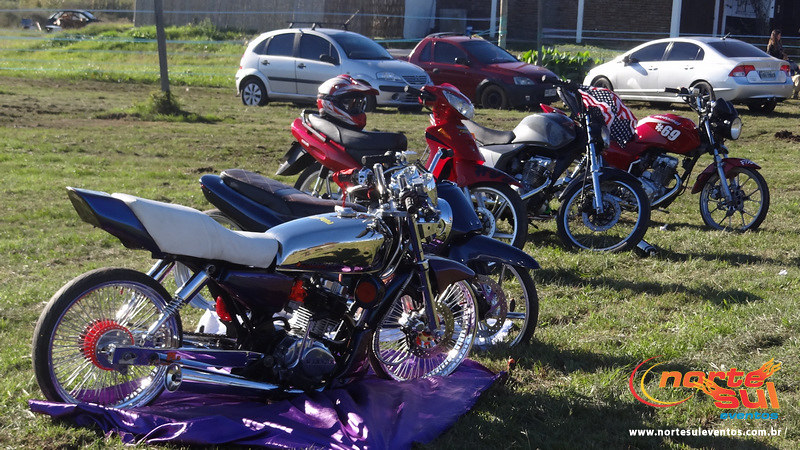This photograph captures a lineup of five motorcycles parked on a grassy field, with a backdrop of three cars and the edge of a building featuring white cylindrical pillars. The first motorcycle in the foreground, positioned on a purple tarp, boasts a gleaming chrome body, chrome rims with mini spokes, and a white leather seat. Behind it, a black motorcycle stands with matching black wheels and seat. The third in line is a red motorcycle with a black seat, on which a red and white helmet is perched. The fourth bike is a gray and black model, decorated with an American flag. The final motorcycle in the row is red and prominently features the number '69' on its gas tank, along with additional chrome elements. All motorcycles are aligned facing to the right, casting long shadows to the right, suggesting the sunlight is coming from the left. In the background, three compact cars—a silver one, a red one, and another silver one—are parked on the grass, oriented in various directions. The image is branded with 'Nortesul' in orange and red text, along with the website 'www.nortesul.com.br,' visible in the bottom right corner.